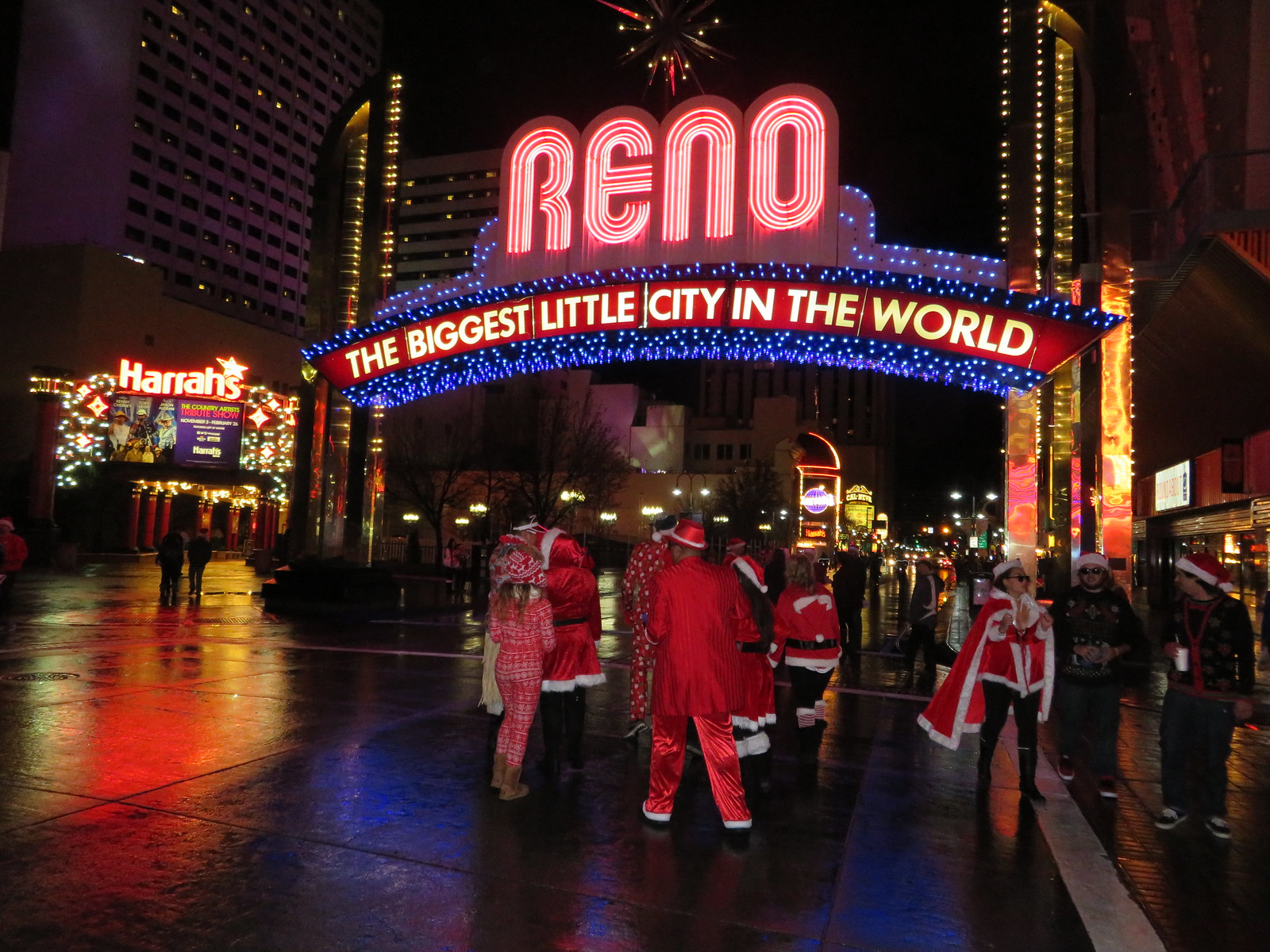This full-color nighttime photograph captures the vibrant and lively scene in downtown Reno, Nevada. Dominating the image, the iconic Reno arch boasts large, bold neon letters spelling "Reno" in red and white, with the tagline "The Biggest Little City in the World" illuminated just below. The street is wet, suggesting a recent rain, adding a reflective sheen that enhances the colorful lights. To the left of the Reno sign, the entrance to Harrah's Casino is visible, with its name lit up and a star marking the apostrophe. Above the Reno arch, a light display, possibly fireworks, adds an extra layer of festivity to the scene. In the forefront, a diverse group of people strolls the busy street, many dressed in Santa Claus outfits with red fabric, black belts, and white fur trims, celebrating what seems to be a Christmas-themed event. One individual stands out in a red satin suit and matching fedora, adding a unique flair to the otherwise festive attire. The background is filled with other illuminated hotels and casinos, completing this electric, holiday-infused atmosphere.